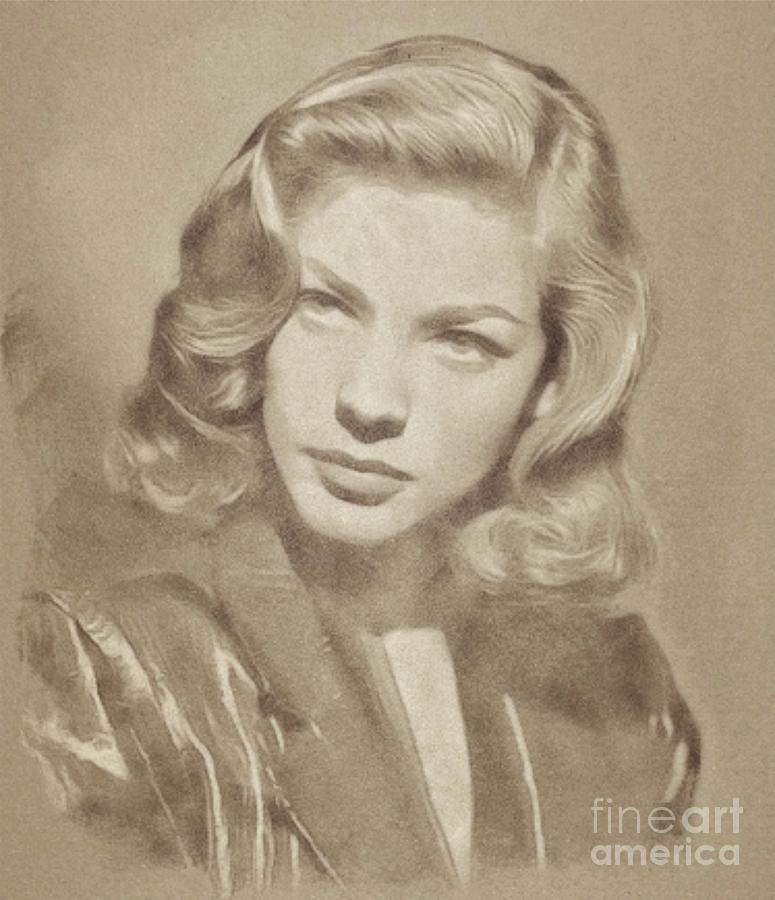This is a digital image of a hand-drawn piece of art depicting the famous actress Lauren Bacall. The portrait, rendered in a realistic style, showcases Bacall from the chest up, adorned in a shiny black outfit that resembles a silk coat with a thick collar, suggestive of 1940s fashion. Her hair, styled in tight, wavy curls reminiscent of the era, cascades just past her shoulders and appears to be a light brown or dark blonde. Bacall's head is tilted upwards towards the top left corner of the image, with her gaze directed in the same direction, capturing a dynamic and thoughtful expression. The artwork employs a monochromatic palette of sepia tones, whites, and beiges, enhancing its vintage aesthetic. The image is signed in the bottom right corner with a watermark that reads "Fine Art America."